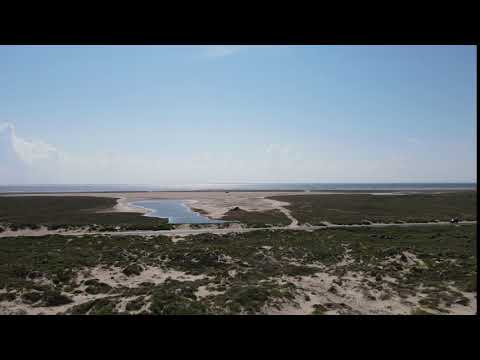The image depicts a photorealistic scene of a beach-like landscape with a small inland body of water, possibly a pond or a small lake, positioned slightly to the left of the center. The photograph, although of relatively low resolution, reveals a combination of sandy and vegetated terrain. In the lower half of the image, the ground alternates between sandy-colored areas and patches of dark green vegetation. A light-colored line, possibly a dirt road, runs horizontally across the image from right to left, interrupting the green patches. Near the waterline, the land appears more sparsely vegetated, with expanses of bare sand. The water in the small pond is a clear blue, and in the background, an expansive body of water, which could be a sea, stretches out towards the horizon beneath a blue sky dotted with small clouds. On the left side towards the bottom corner, there is a large, prominent white cloud. The distant flatness of the landscape gives an impression of an endless horizon, enhancing the serene, open atmosphere of the scene.